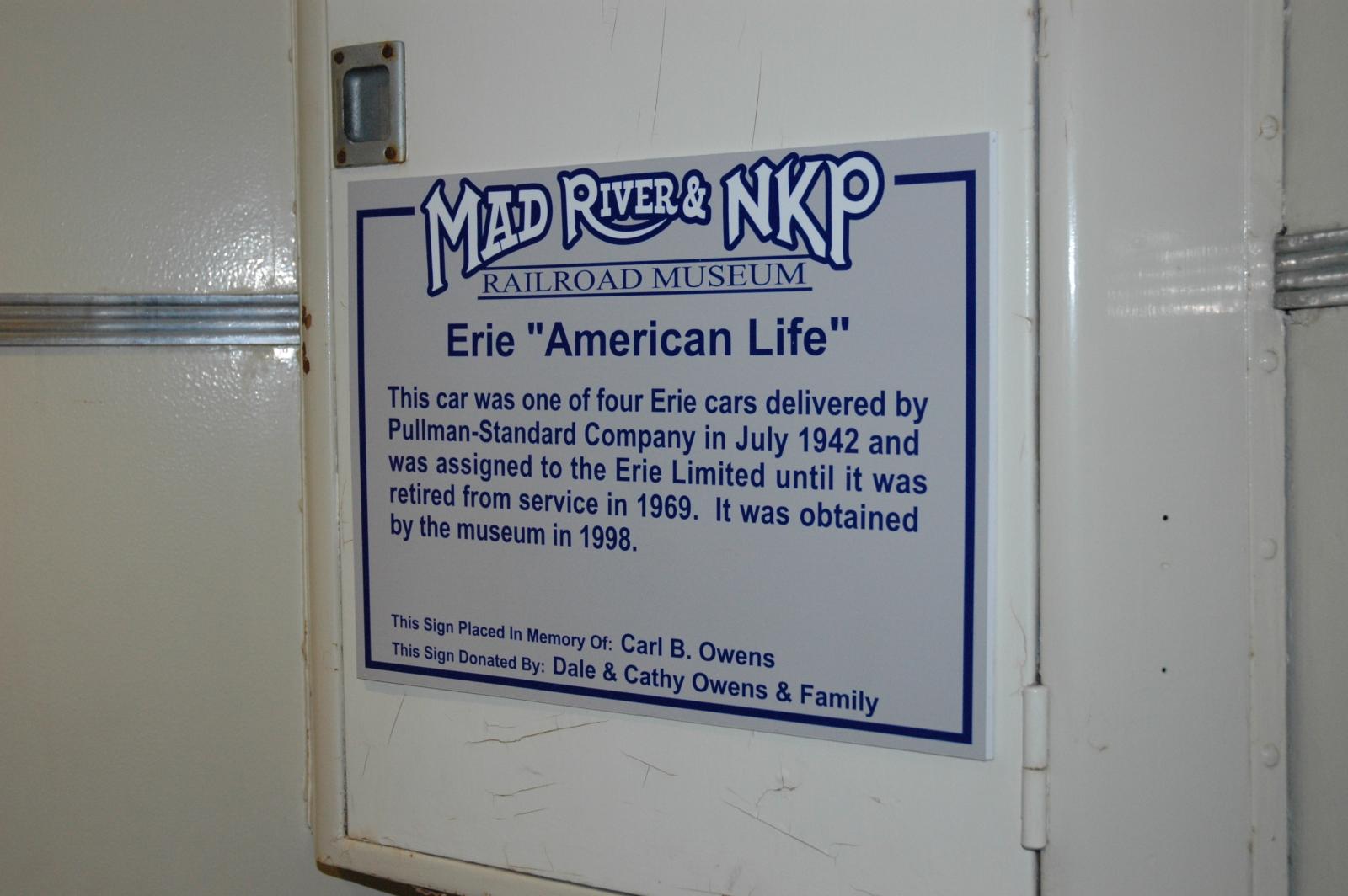This detailed color photograph shows a sign affixed to a large, white metal box that is mounted on the interior wall of a railroad car, located at the Mad River and NKP Railroad Museum. The sign itself features a gray background with a blue rectangular border and blue text. At the top, in white text with a blue border, it reads "Mad River and NKP Railroad Museum." Below that, in larger blue letters, it says, "Eerie American Life." The placard further details that this car was one of four "Eerie" cars delivered by the Pullman Standard Company in July 1942 and was assigned to the Eerie Limited until its retirement from service in 1969. It notes that the car was obtained by the museum in 1998. At the bottom, it reads, "This sign placed in memory of Carl B. Owens," and states that the sign was donated by Dale and Kathy Owens and family. The image captures additional details such as metal conduits extending from the left and far sides of the box, a metal handle near the top of the box door, and hinges on the right side, indicating it is likely an electrical box. The background shows part of a white wall, potentially at a corner, enhancing the indoor setting of the photograph.